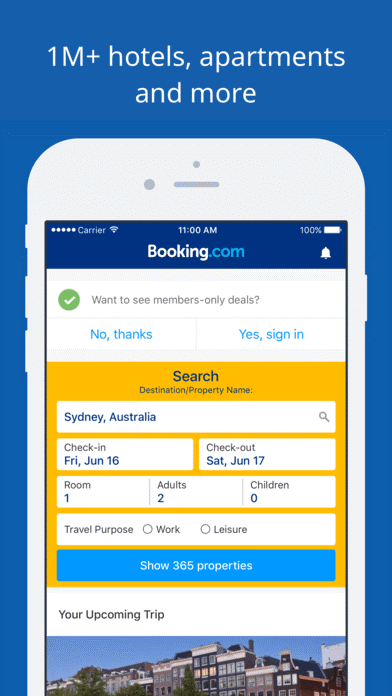The image is a portrait-style, royal blue rectangular advertisement for Booking.com. At the top, white text boldly announces "1M+ hotels, apartments, and more." Beneath this text, a smartphone is prominently displayed with the Booking.com website open on the screen. The website features a dark navy header with a prominent Booking.com logo. Below the header, there is a white block containing a green circle with a white arrow, accompanied by the text "Want to see members-only deals?" followed by two options: "No thanks" and "Yes, sign in."

Further down, the website's search feature is highlighted within an orange block, where the search field displays "Sydney, Australia" as the destination. The check-in date is set for Friday, June 16th, and the check-out date is Saturday, June 17th. The reservation is for one room, accommodating two adults with no children, and specifies no travel purpose, whether for work or leisure. There is also a blue block with white text that reads "Show 365 properties." Below this, the beginning of a section titled "Your upcoming trip" is visible, partially revealing a photograph of buildings.

Overall, this advertisement effectively promotes Booking.com by showcasing the user-friendly interface and highlighting the ease of making travel reservations.